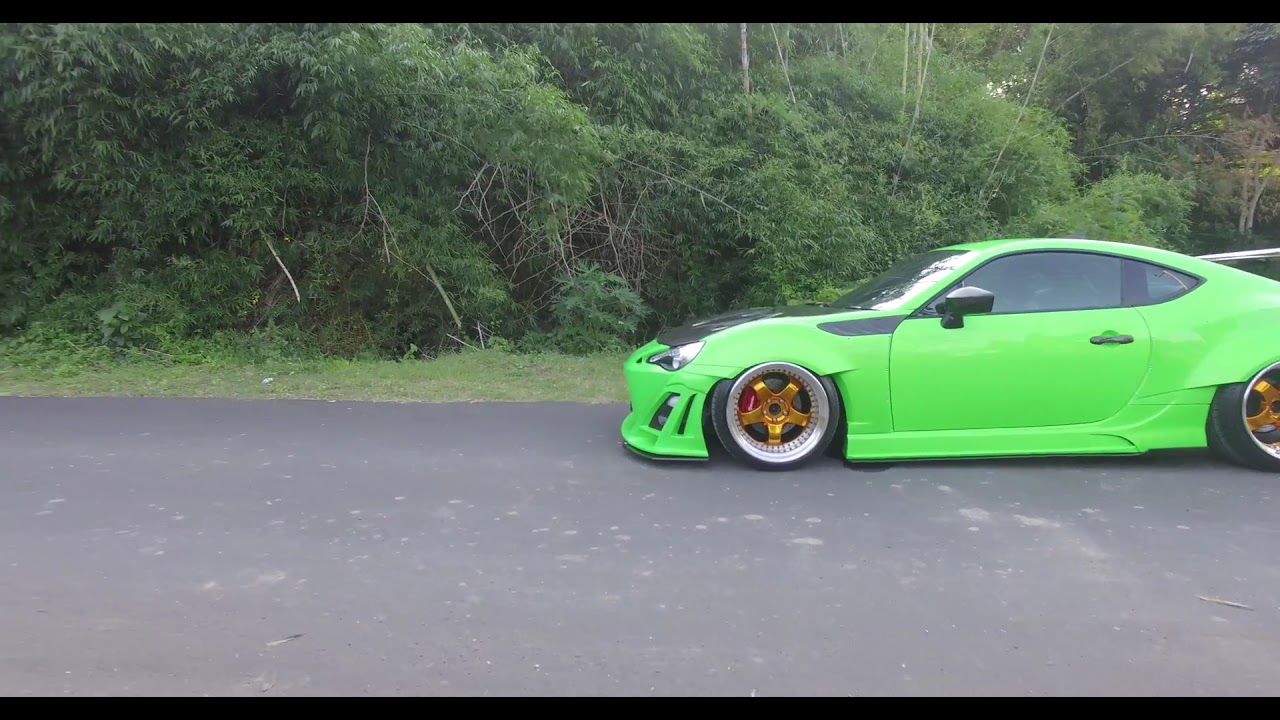The image features a vibrant neon green, two-door sports car positioned on the right side of the frame, extending towards the middle. The car stands out with its striking modifications, including gold starfish-shaped spokes in the center of the rims, which are encircled by a silver outer ring. The low chassis of the car hugs the clean, dark gray asphalt road, creating a stark contrast with the lush, dense backdrop. The road, although slightly marred by splotches of dirt, appears well-maintained. The background showcases a thick wall of impenetrable vegetation comprising numerous green bushes, slender tree trunks, and branches. The photograph, framed with a thin black header and footer, has an elevated vantage point of about six feet off the ground, capturing the surreal juxtaposition of the almost cyberpunk-like car against the earthy, natural surroundings. The car's tinted windows obscure the interior, hinting at, but not clearly revealing, a possible driver within. The image dramatically cuts off around the car's back tire, leaving the full extent of the vehicle unseen.